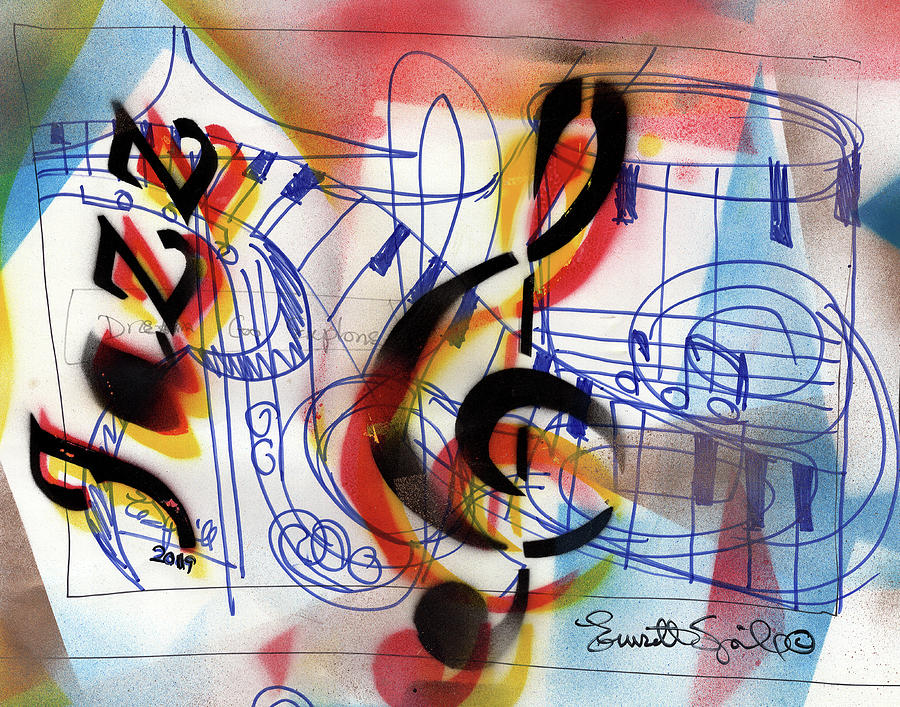This abstract artwork features a dynamic blend of colors and musical themes on a predominantly white background. The upper portion is dominated by vibrant red and yellow hues forming shapes reminiscent of musical symbols, alongside a distinct black music note that curls gracefully into an S-shape. These elements seem to overlay or shadow each other, creating a layered effect. On the left side, the letters "J-A-Z-Z" are creatively arranged in black, red, and yellow, oriented vertically and slightly rotated. Blue-inked musical elements, including crudely drawn piano keys, provide a textured background that spans across the image, especially noticeable in the bottom right corner. Here, you will also find the artist's signature inscribed in black cursive, with a horizontal line extending from the signature across the image. However, much of the text and musical notes underneath the overlay are indecipherable. The piece merges traditional artistic techniques with digital flair, creating a vibrant homage to music.